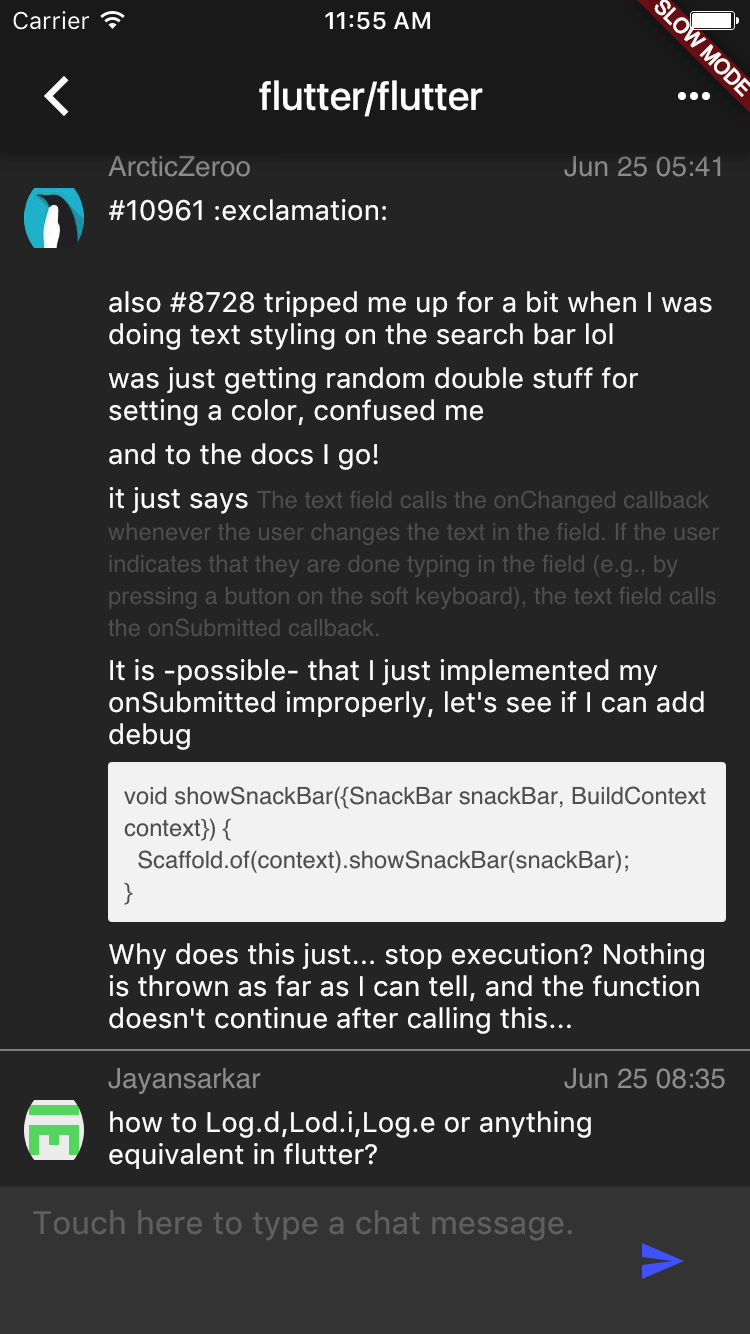**Screenshot Description**

The image is a screenshot from a phone using dark mode, showcasing white text against a black background.

**Top Bar:**
- **Upper Left Corner:** The word "Carrier" is displayed with the Wi-Fi signal strength icon next to it.
- **Upper Center:** The time is shown as "11:55 AM."
- **Upper Right Corner:** A white battery icon appears, along with a red ribbon labeled "Slow Mode."

**Left Section:**
- Beneath "Carrier," there's a white right arrow icon pointing to the left.

**Main Body:**
- The center of the screen prominently displays "flutter/flutter" followed by three dots.
- Below this, a section with a lighter gray background begins.

**Gray Section:**
- **Left Side:** A blue circle containing a cartoonish penguin facing left, labeled "Arctic Zeroo" (with an extra 'O').
- **Right Side:** Displaying the date "June 25" and the time "05:41."
- Below this, some additional textual information includes:
  - "#10961" followed by a descriptive explanation about troubleshooting text styling issues:
    ```
    #8728 tripped me up for a bit when I was doing text styling on the search bar, LOL. Was just getting random double stuff for setting a color, confused me. To the docs I go!
    ```
  - An explanation about text field callback behavior:
    ```
    The text field calls the onChanged callback whenever the user changes the text in the field. The user indicates that they are done typing in the field, e.g., by pressing a button on the soft keyboard, and the text field calls the onSubmitted callback. It is possible that I just implemented my onSubmitted improperly. Let's see if I can add debug.
    ```

**Method Description:**
- A white box contains the definition of a method:
  ```
  void showSnackBar(SnackBar snackBar, BuildContext context) {
    Scaffold.of(context).showSnackBar(snackBar);
  }
  ```
- Below this, there is a query:
  ```
  Why does this just stop execution? Nothing is thrown as far as I can tell, and the function doesn't continue after calling this...
  ```

**Additional Conversations:**
- A thin gray line divides sections.
- **Left Side:** An icon of an upside-down green 'E' inside a white circle and the name "JAYANSARKAR."
- **Right Side:** The date and time "June 25, 08:35."
- Below this, there is a question about logging in Flutter:
  ```
  How to log.d, log.i, log.e, or anything equivalent in Flutter?
  ```

**Input Box:**
- At the bottom, a text box prompts:
  ```
  Touch here to type a chat message.
  ```
- An adjacent blue arrow points to the right.